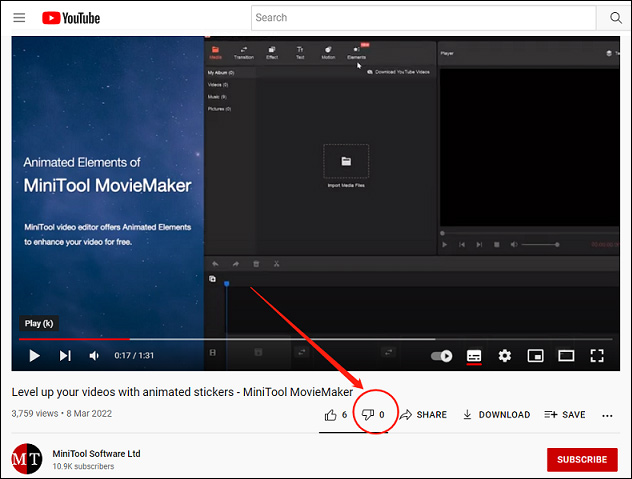The image is a YouTube screenshot displaying the user interface prominently. At the top-left corner, the YouTube logo is displayed next to the menu icon, followed by the search bar. Below this, a video thumbnail catches the eye with text reading, "Animated Elements of MiniTool Movie Maker." The video highlights that MiniTool Video Editor offers animated elements to enhance your videos for free. To the right of the thumbnail, there is a visual depiction of the editor in action. A red arrow points from the video thumbnail to a circled thumbs-down icon, which currently shows zero dislikes.

Beneath the thumbnail, the video is titled "Level Up Your Videos with Animated Stickers - MiniTool Movie Maker," and has garnered 3,759 views since its upload on March 8th, 2022. The video's uploader is identified by a profile picture with the initials "MT" and the name "MiniTool Software LTT," boasting 10.9K subscribers. A "Subscribe" button is prominently placed in the lower right-hand corner.